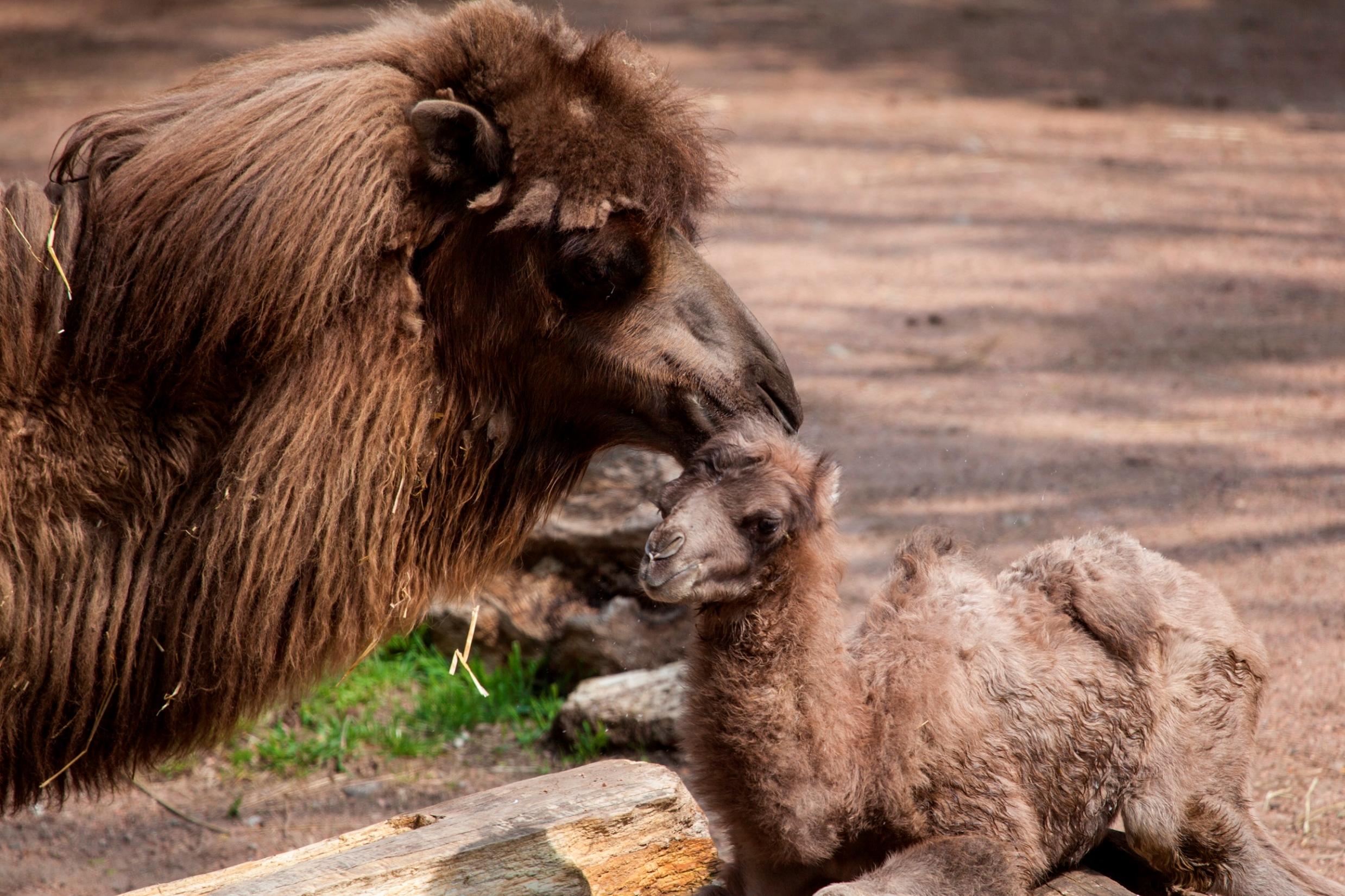This is a close-up, horizontal color photograph taken in a seemingly artificial desert-like setting, possibly a zoo. It captures an intimate moment between two long-furred Asian camels. The central figures are a mother camel and her baby, both adorned with shaggy brown fur. The mother's fur is darker and longer, with tufts and debris embedded in it, while the baby's fur is fluffier and a lighter shade of brown.

The mother camel, positioned on the left, has her head and neck prominently featured, extending towards the center of the image where she appears to be gently kissing or grooming the baby camel. Her large, expressive eyes, stubby ears, and long muzzle are clearly visible. She exudes a protective and caring aura.

The baby camel lies on the ground, occupying the bottom right of the image. Its long snout, black eyes, and small ears enhance its endearing appearance. The baby's small patch of green grass and scattered rocks next to a wooden log in the foreground adds a touch of natural texture, contrasting with the otherwise sandy, dirt-brown background.

The overall atmosphere of the picture is tender and serene, capturing the bond between mother and offspring in an intimate and detailed manner.